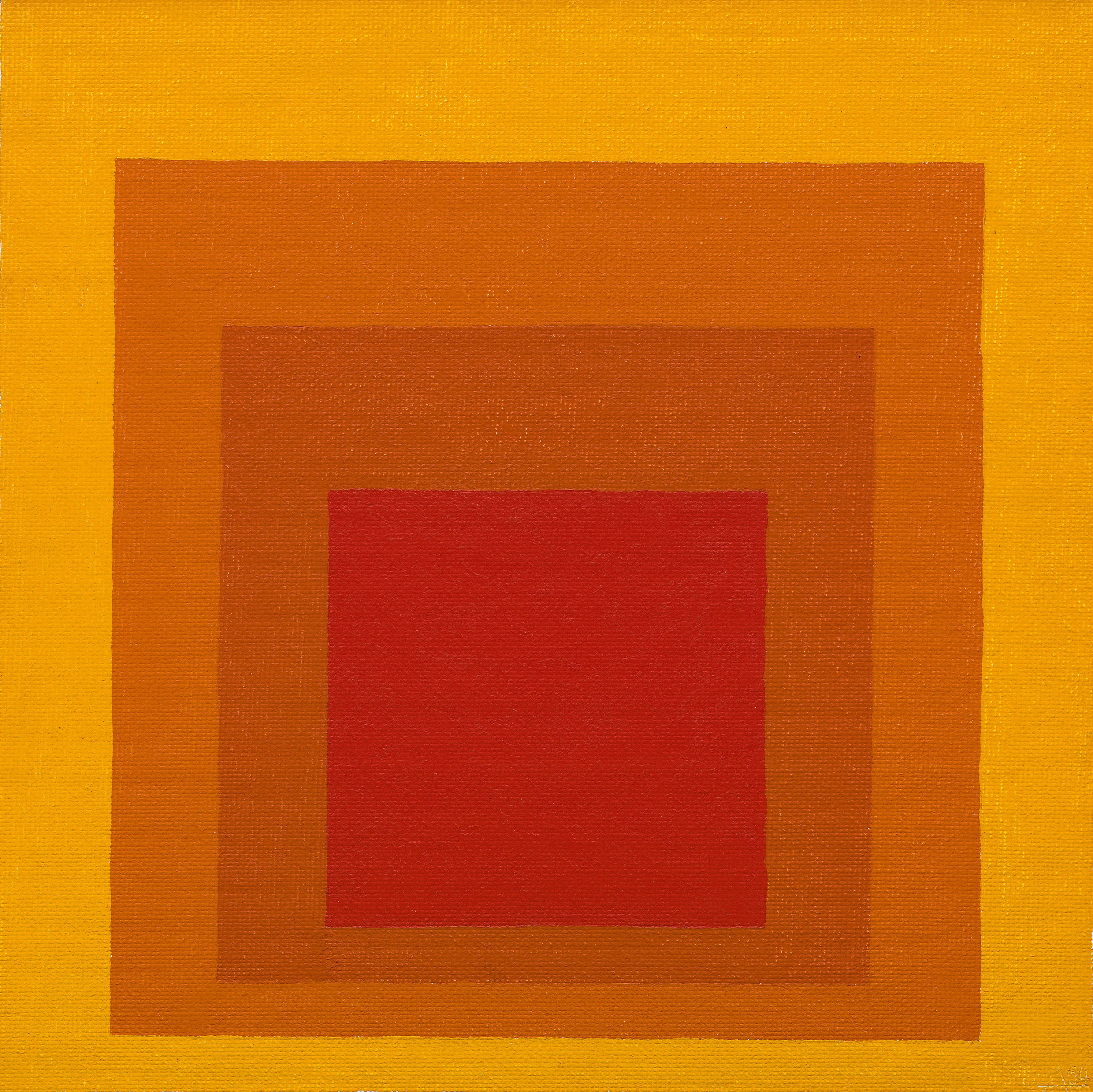The image depicts an abstract painting reminiscent of Mark Rothko's style, characterized by a composition of nested squares that evoke the impression of a color gradient. At the center of the artwork is a brick red square, which is then surrounded by a progressively larger brown frame. Encasing these is an orangey hue, finally bordered by a golden ochre yellow outermost square. The overall effect creates a layered appearance, akin to a series of frames or a nested Russian doll. The piece is devoid of any text or background context, focusing solely on the interplay of simple, bold colors. The artwork is unsigned, yet clearly invokes the mid-20th century modernist aesthetic that is often associated with Rothko's iconic, large-scale abstract paintings.